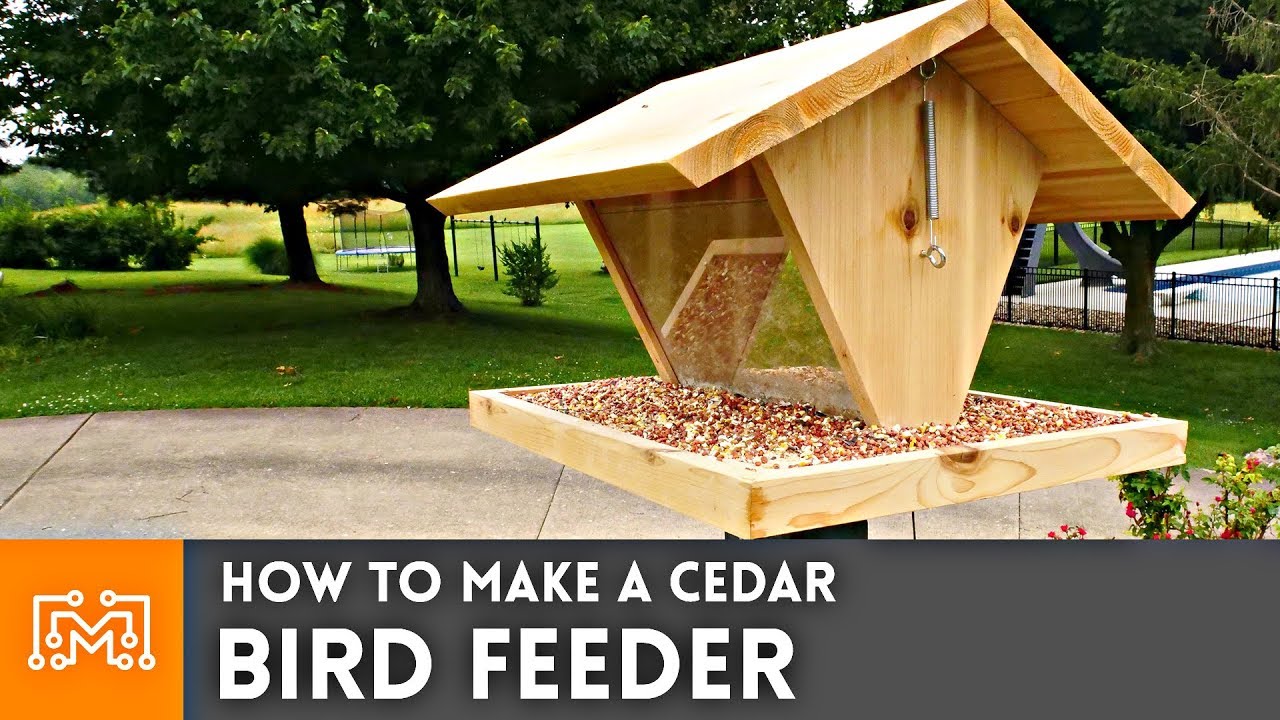This horizontal ad features a detailed image of a cedar bird feeder prominently displayed in a lush, outdoor setting. The bird feeder stands at the center, surrounded by vibrant green grass, various bushes, and colorful red or pink flowers with green leaves. The background is filled with trees showing a mix of green and yellow foliage, and some branches and stems are visible, appearing brown. To the right, a pool with blue water and a gray slide is bordered by a white sidewalk and a mix of tan, white, and black rocks. The bird feeder itself is designed to look like a house with a brown base, a tray filled with bird feed, and glass windows on either side. It is mounted on a black post and includes a silver metal component hanging from its side. Below the image is a gray banner with white, all-caps text that reads "HOW TO MAKE A CEDAR BIRD FEEDER." To the left of this text, an orange square with an 'M' in white is featured, possibly representing a logo. This visually rich scene suggests a serene backyard, making the bird feeder and the instructional content below it the focal points of the advertisement.